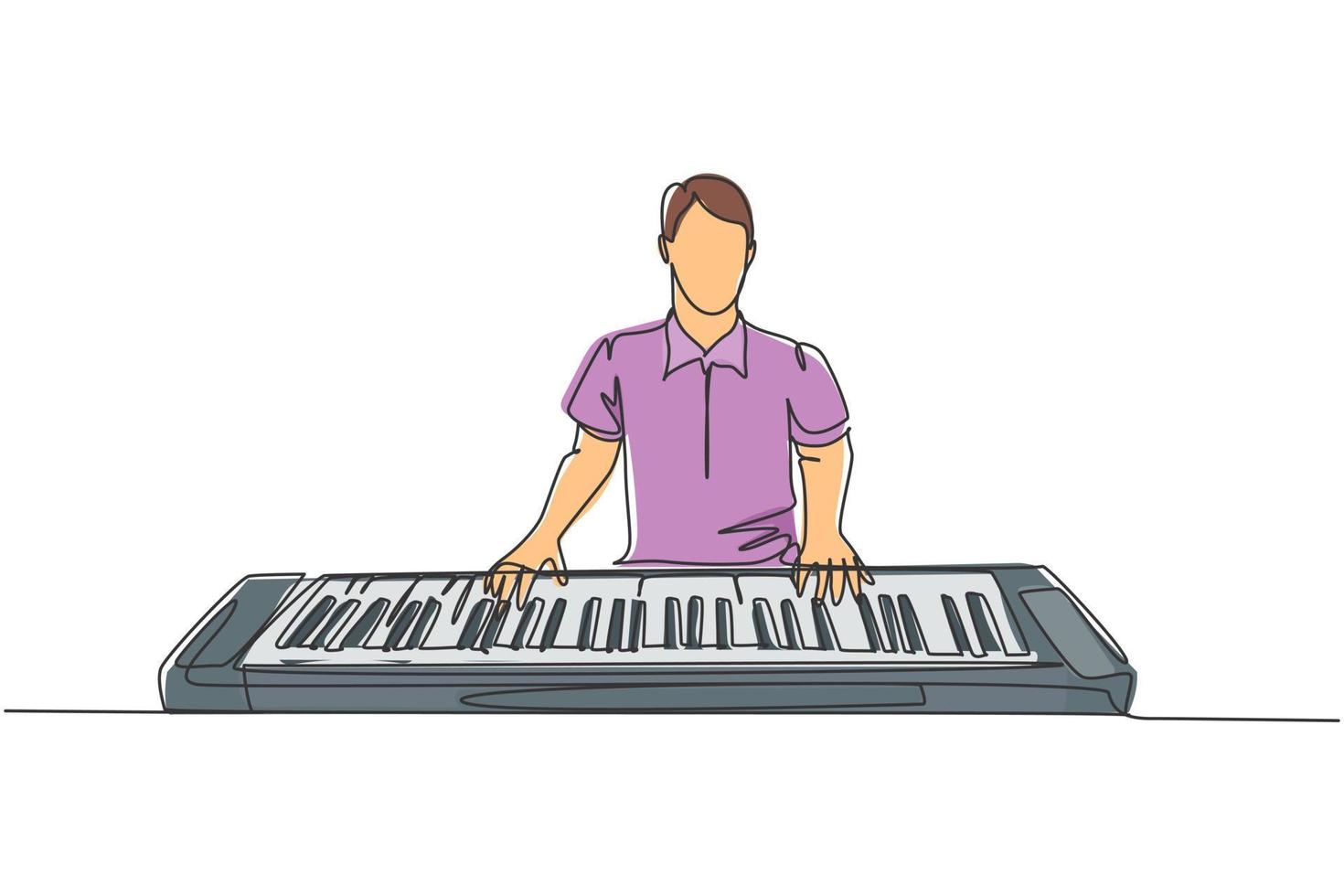This image is a detailed cartoon illustration of a man with light skin and brown hair, combed to the side, playing a synthesizer. He is donned in a short-sleeved, purple collared shirt resembling a polo style. The man’s face is featureless, giving him a blank expression. The synthesizer he is playing is predominantly gray with both white and gray keys, though there is a mention of black keys, suggesting variations. His arms and hands appear detached from the keyboard, seemingly clipping through the instrument in a manner that suggests a stylistic choice, perhaps indicating the image was drawn with a continuous line technique. The background is entirely white, providing no additional context or detail. The overall appearance of the illustration is somewhat minimalistic and abstract, contributing to a somewhat unfinished or conceptual feel.